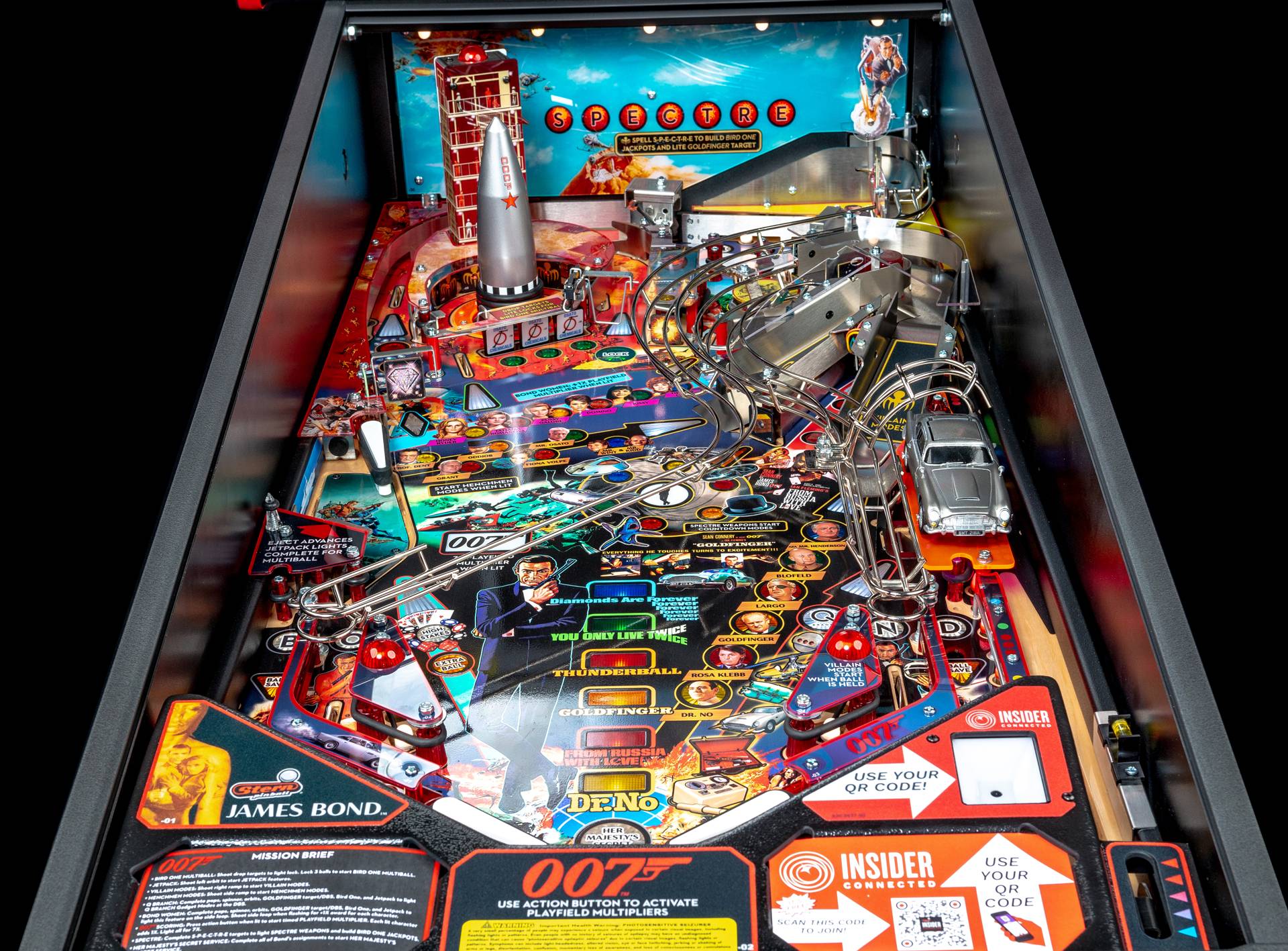The image is a zoomed-in, detailed aerial view of the inside of a vibrant old 007 James Bond pinball machine. Featured prominently is an illustrated depiction of Sean Connery in the iconic James Bond pose, holding a gun. To the right of Bond, several classic villains such as Dr. No and Oddball are illustrated. There is also a silver Aston Martin, the quintessential vehicle Bond drives, positioned just above the rail where the ball gets fired. In the top left corner, a missile adorned with a red star—likely a reference to a Russian nuke from Goldeneye—can be seen. The word "SPECTRE" is featured in the background, with each letter encased in its own circle. The colorful playfield includes various hues like blue, red, green, orange, and white, adorned with directional arrows that guide the gameplay. Some arrows have small inscriptions, such as a red arrow stating "use your code" and a green one marked "insider," although some words remain too small to identify. The scene is vibrant and bustling, encapsulating the thrilling essence of James Bond's cinematic adventures.